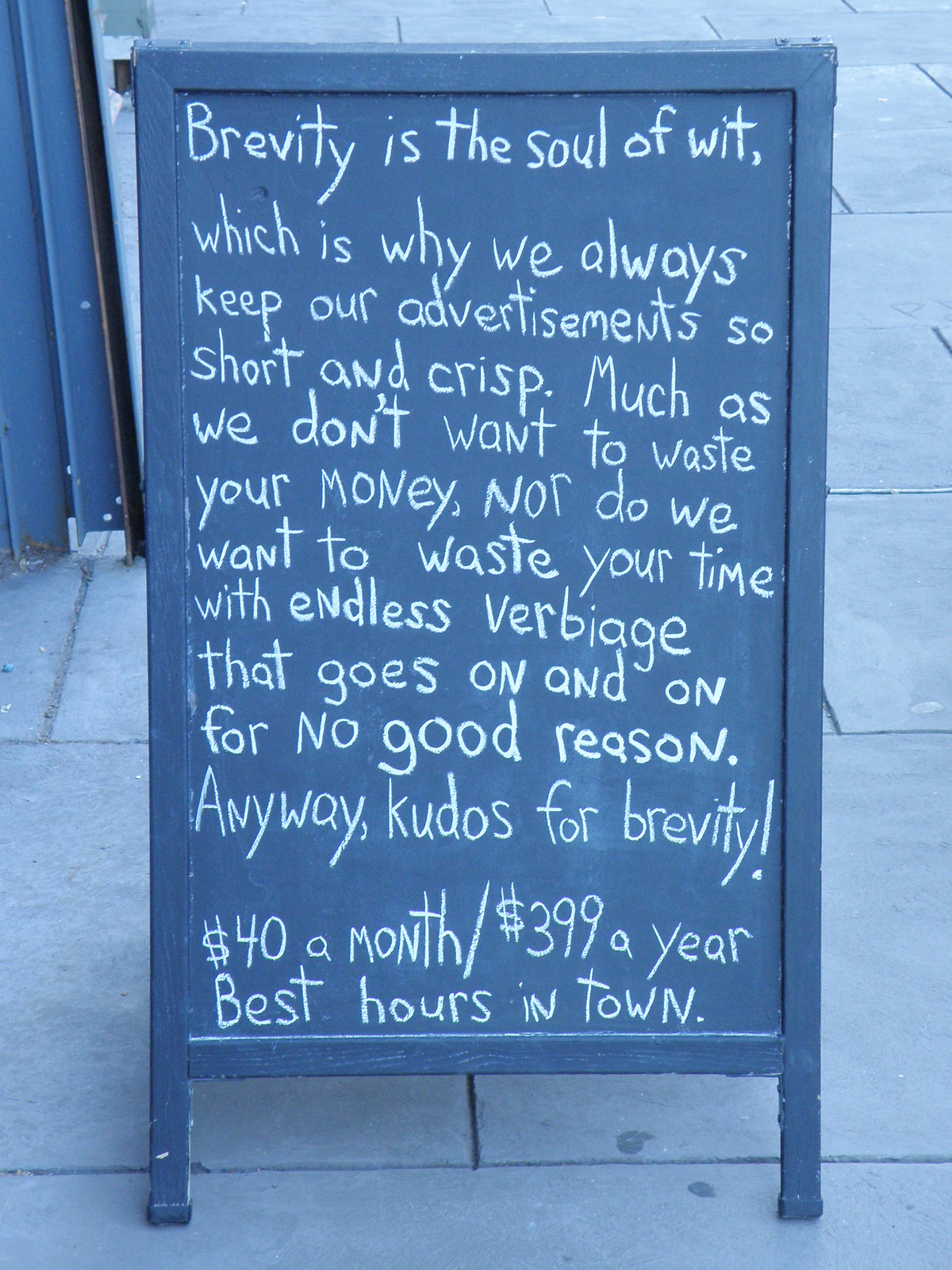The photo shows a propped-up chalkboard sandwich board on a stone-tiled sidewalk, possibly in front of a blue-painted building partially visible in the upper left corner. The sign, set in a green wooden frame, features white chalk text that reads: "Brevity is the soul of wit, which is why we always keep our advertisements so short and crisp. Much as we don't want to waste your money, nor do we want to waste your time with endless verbiage that goes on and on for no good reason. Anyway, kudos for brevity. $40 a month, or $399 a year, best hours in town." This humorously sardonic advertisement ironically comments on the value of brevity while promoting a service, although the specific business is not identified.